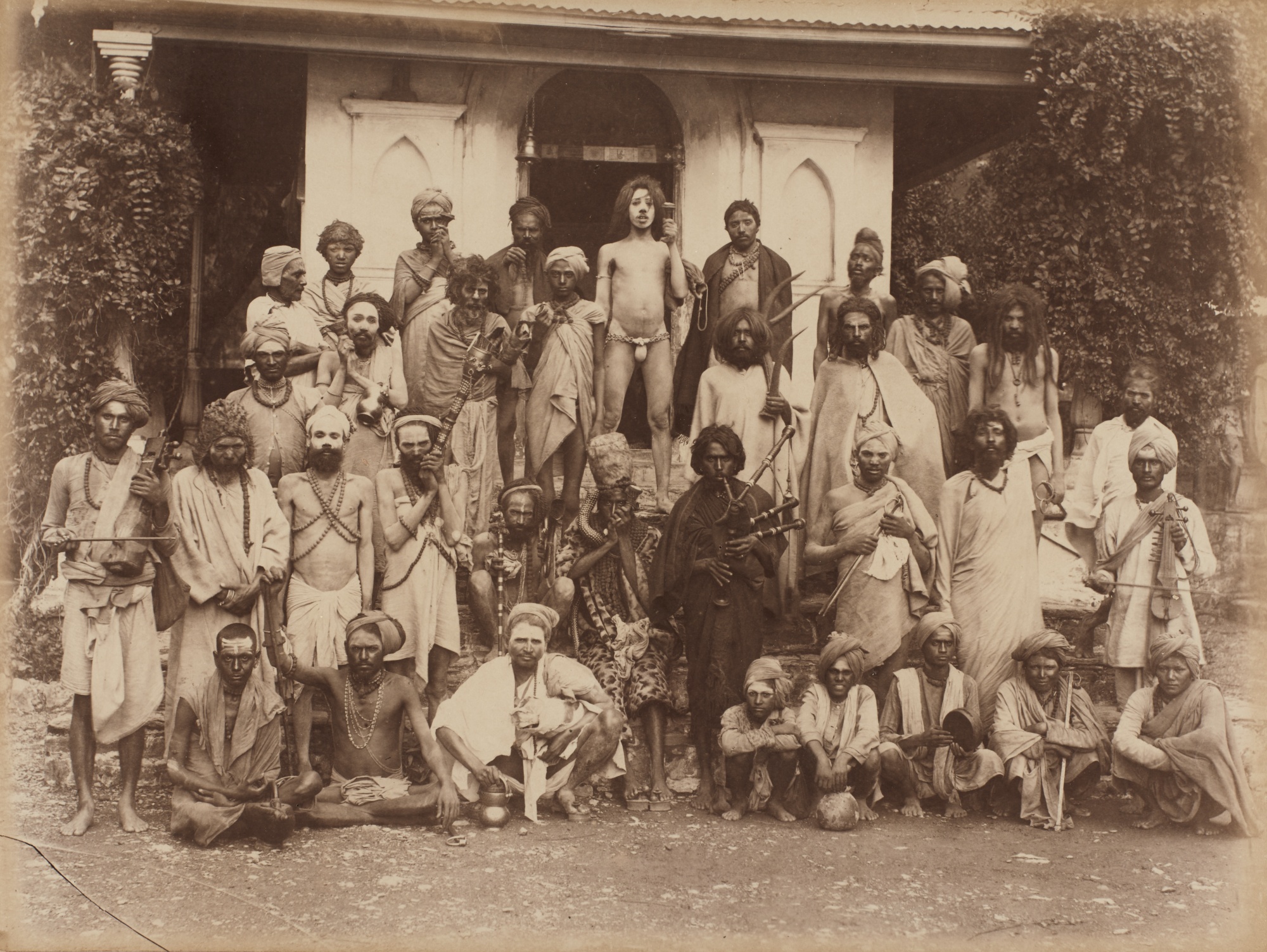The black-and-white vintage photograph depicts a large group of men arranged in a triangular formation outdoor. They stand against the backdrop of dark trees and a white stone column, suggesting a structured environment. Men in the front row are seated, while those in the middle stand at ground level, and the rear row stands on higher ground or steps, culminating with one individual at the very top. Many of the men wear head turbans, robes, and wrapped skirts, exuding a tribal or indigenous appearance. Their skin appears dark, possibly accentuated by white paint on their foreheads. Some men seem bound by chains and hold weapons, hinting at a sense of unrest or captivity. The photograph bathes in natural light, offering a bright and clear view of the scene.